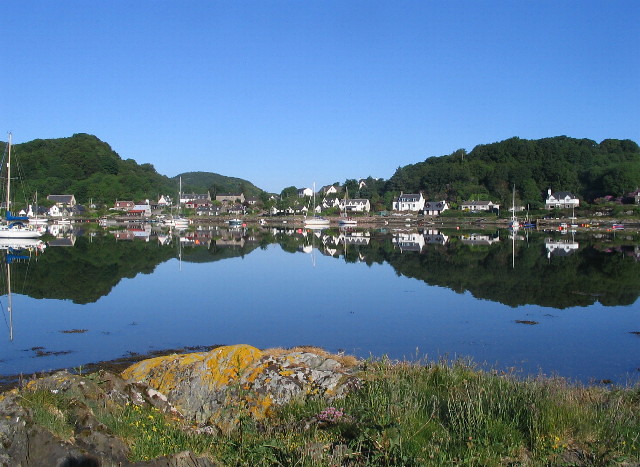The photograph captures a serene scene of a small village nestled on the edge of a tranquil bay, possibly along the east coast. The landscape orientation image shows a wide view taken from afar, revealing an expanse of reflective, still blue water that mirrors the vibrant blue sky above and the healthy green trees lining the shore. In the foreground, there's an abutment of land dotted with dark green foliage and patches of gold moss, along with some sparse, reed-like grass and a prominent rock.

Across the bay, a cluster of clean, well-kept boats are moored at the dock, and several large buildings stand alongside smaller ones, all predominantly white with dark gray roofs. These structures extend along the shoreline. The entire village rests against two small hills with more expansive, tree-covered mountain ranges visible in the background. The calm water perfectly reflects the buildings and the lush greenery, adding to the picturesque and idyllic charm of the scene.